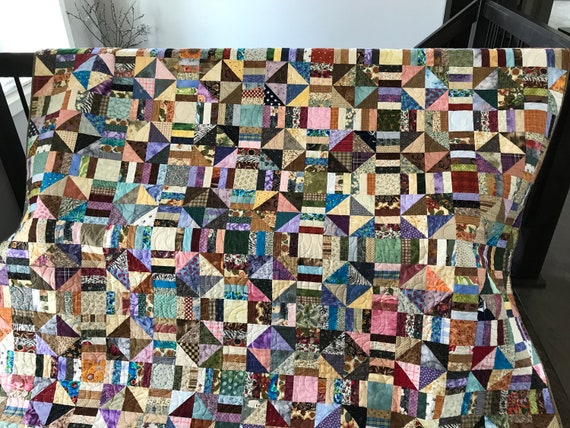The photograph features a detailed, handcrafted quilt prominently displayed, draped over what appears to be a black wooden bench or child fence in a room with white walls partially visible in the background. This multi-colored quilt is composed of numerous one-inch-by-one-inch fabric squares, intricately stitched together in a patchwork design. The squares exhibit a blend of vibrant colors including shades of pink, purple, yellow, brown, and blue, each with unique fabric patterns. These small squares form a distinctive diagonal pattern, creating a diamond shape when grouped in fours. A hint of a plant can be seen peeking out in the upper left corner of the image. The artistic craftsmanship and precise arrangement of the squares suggest that, although quilted, the piece may also serve as a decorative wall hanging. The quilt appears to be two feet by three feet in size and is positioned in such a way that it occupies the central focus of the photograph.